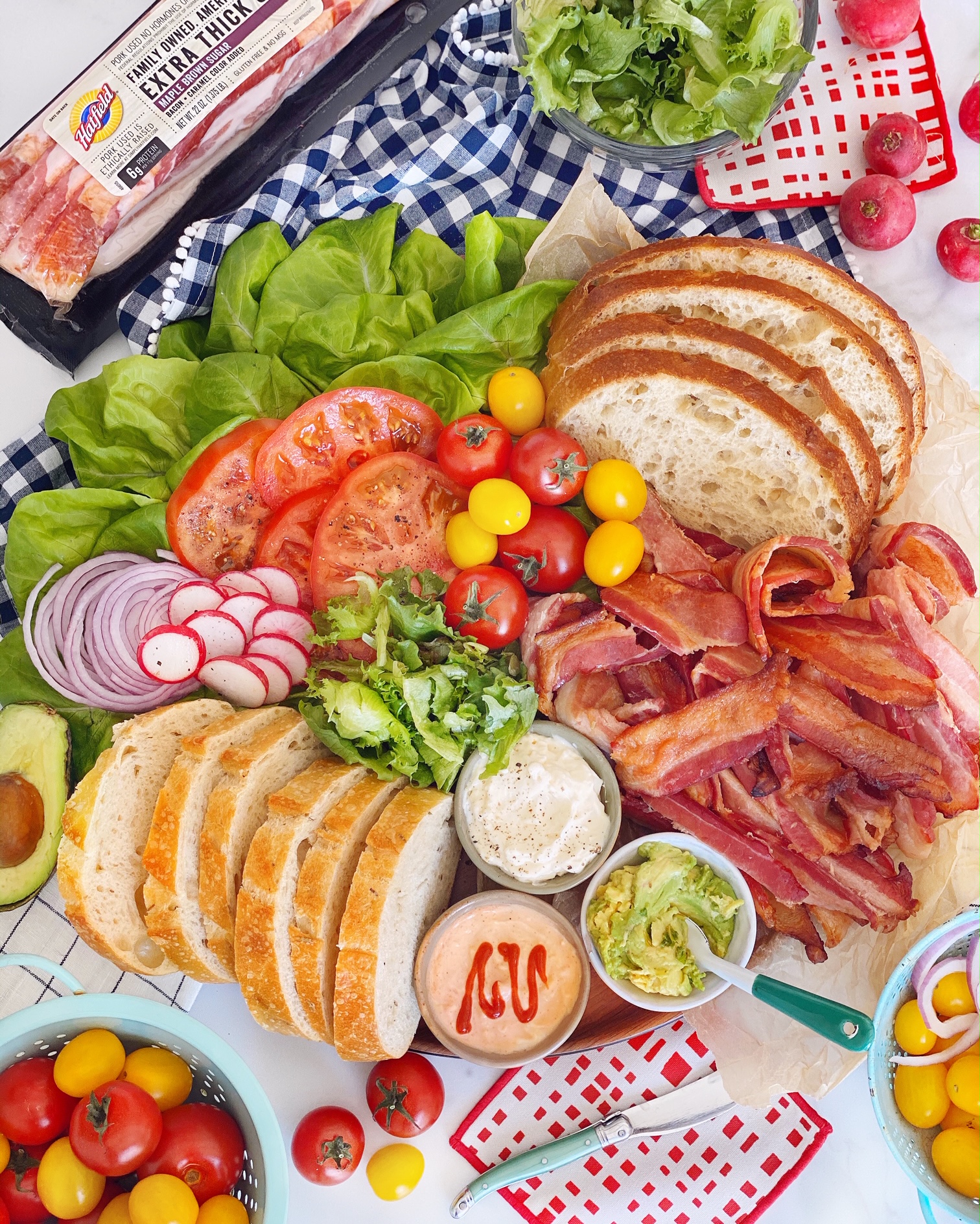This detailed, overhead photograph showcases an extensive spread for preparing BLT sandwiches, laid out on a white and blue checkered tablecloth. At the top of the image, a package of extra thick bacon from Hatfield is prominently displayed, hinting at the mouthwatering, cooked bacon piled just in front of sliced bread on a bed of fresh lettuce. The arrangement features both whole and halved cherry tomatoes, some in vibrant yellows and reds, thoughtfully placed in blue colanders. Surrounding these are neatly sliced tomatoes, onions, radishes, and accompanying leafy greens, including spinach and assorted lettuces. Additionally, three small cups of sauces—possibly guacamole, ranch, and an aioli—add to the variety, each with distinct colors: green with a spreader spoon, an orange-tinted one with red streaks, and a white, creamy option. Nestled to the side, a bowl holds more cherry tomatoes, next to a halved avocado and a collection of colorful, checkered potholders in red and white. This inviting presentation sits atop what appears to be a tiled cutting board, ready for the sandwich assembly process.